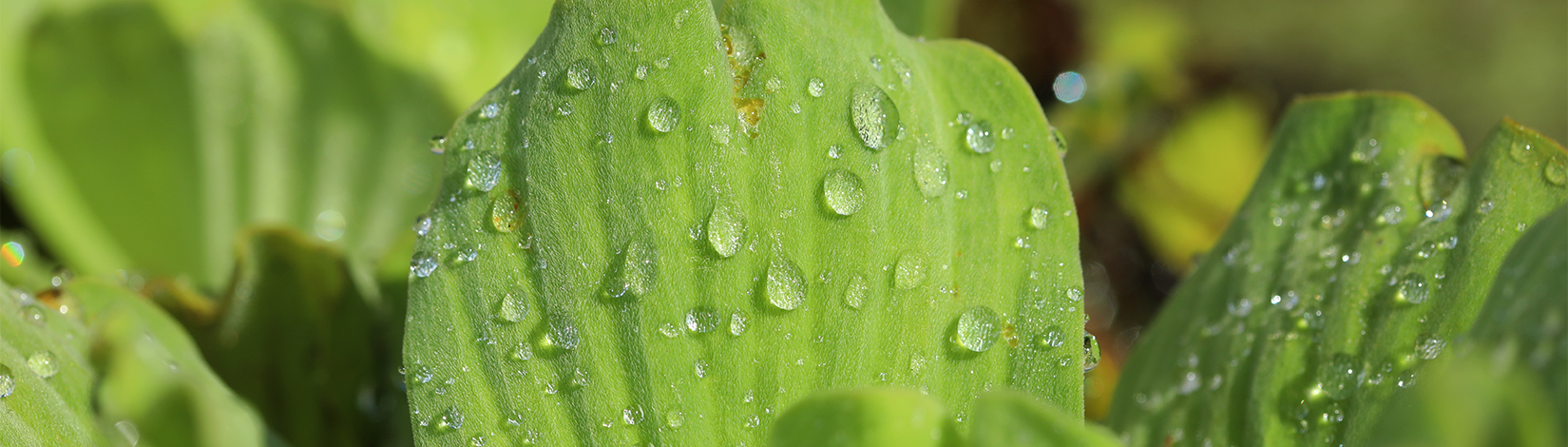This photograph captures a wide, narrow, panoramic close-up of brightly colored green leaves, predominantly featuring one leaf that is coated with numerous small, spherical water droplets. The teardrop-shaped droplets, which may be the result of recent rain or dew, glisten in the sunlight, suggesting a fresh, sunlit day. The leaves have broad surfaces with small ridges, and while the primary focus is sharp and detailed, the background fades into a blurry mix of similar leaves, enhancing the sense of depth without introducing any distinct shapes. Despite the clarity of the central leaf, the plant species remains unidentified. The overall scene conveys a feeling of freshness and natural beauty, accentuated by the intricate interplay of light on the water droplets.